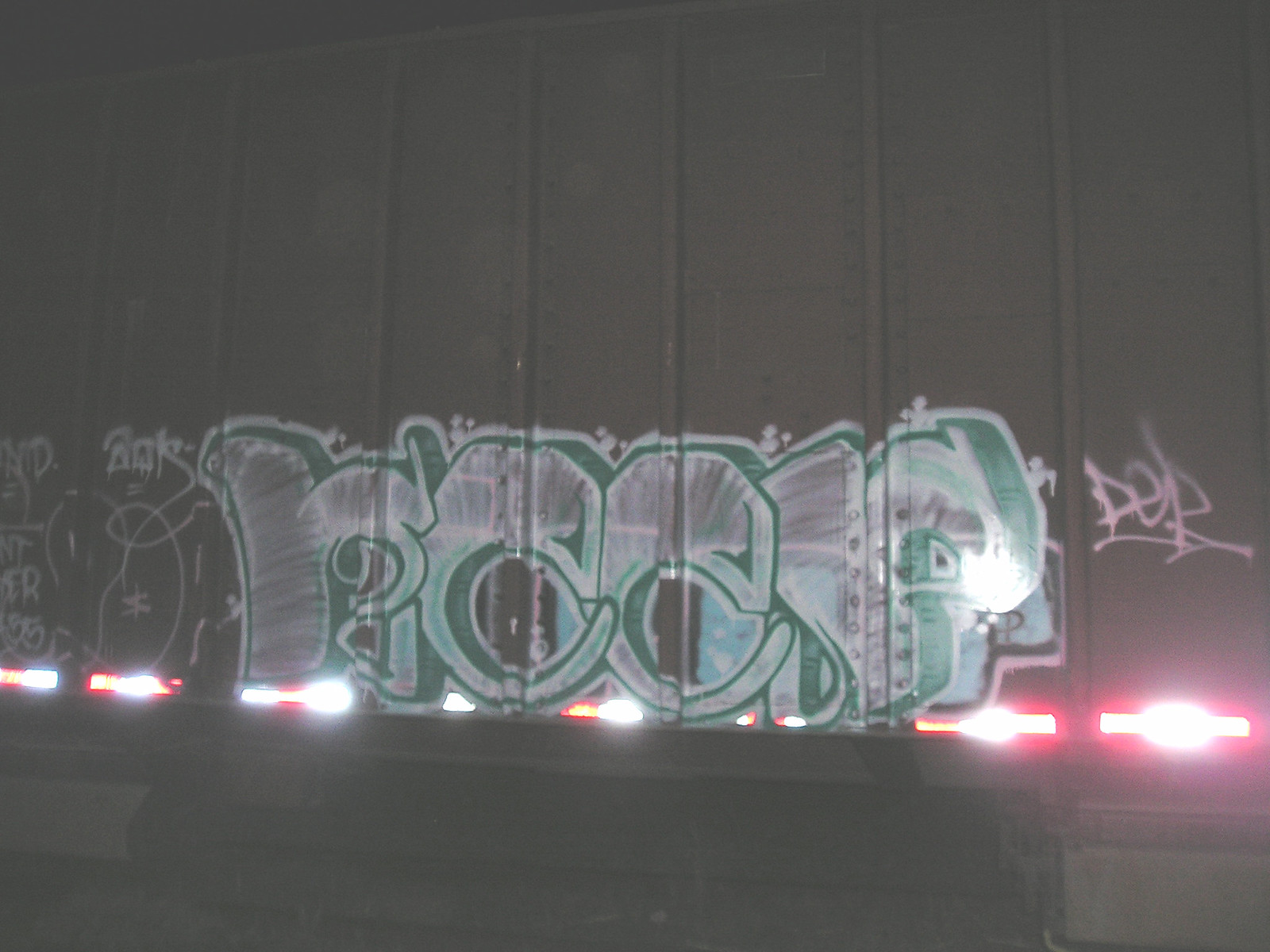This photograph captures an intricate display of graffiti adorning a dark gray railroad tank car. The tank car features vertical and horizontal support lines running across it. Illuminating the scene are bright lights concentrated on the right side, transitioning from a white light in the center to an orange halo around it, shifting to a lit-up orange hue as they move leftward.

Above these lights, the graffiti is prominently showcased in white and green spray paint. The primary design consists of white letters outlined in green, potentially forming the letters "R C C P," though the exact wording is somewhat ambiguous. Adjacent to these letters on the right, the characters "P E P" are discernible in white spray paint.

On the far right side, there's a signature in white spray paint, while the far left side features random white spray paint drawings. Additionally, the left section of the tank car displays a banana-like shape sloping leftwards with an indistinct character in its center. Further to the left, there are two interlinked shapes resembling handcuffs, mirrored by another unidentified design on the right side. The photograph appears to have been taken at night, adding to the dramatic illumination of the graffiti.